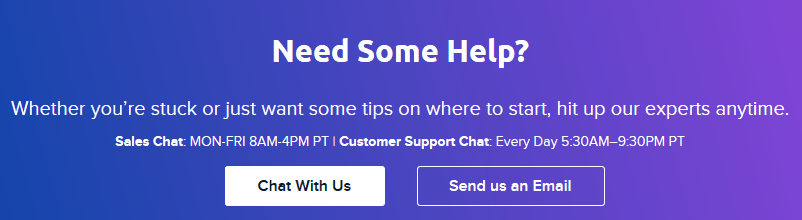The image features an elongated rectangular gradient background transitioning from a dark blue-tinted violet on the left to a lighter, brighter violet on the right. At the top, bold, white, sans-serif font text reads, "Need some help?" Below, slightly blurry white text, indicative of a low-quality image, states: "Whether you're stuck or just want some tips on where to start, hit up our experts any time."

Further down, in a small white bold font, it says "Sales Chat:" followed by non-bold text, "MON-FRI 8 AM-4 PM PT." 

A divider separates this from the next section, which in bold reads, "Customer Support Chat:" followed by non-bold text, "Every day 5:30 AM-9:30 PM PT."

At the bottom, there are two rectangular call-to-action buttons. The left button, with rounded edges and a white background, displays "Chat with us" in bold black lettering. The right button, featuring a transparent background that blends into the gradient, has a white border and rounded corners, and says "Send us an email" in bold white text.

The top section occupies a significant vertical space before the headers begin, implying a balanced and spacious layout. The entire design is clean and organized, encouraging interaction with the provided support options.